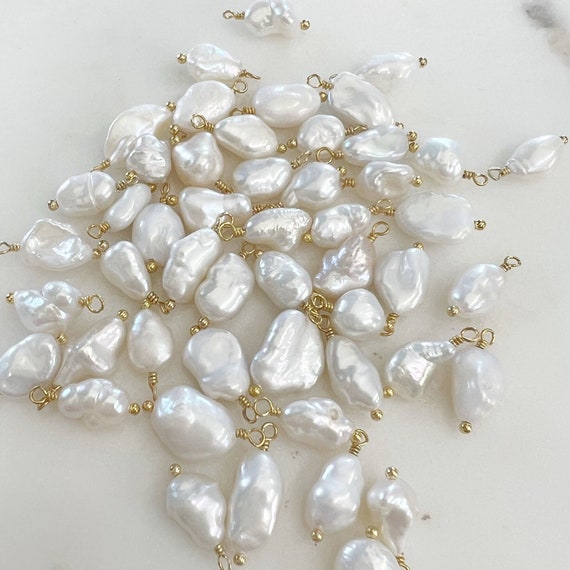This is an overhead photo capturing dozens of irregularly shaped pearl-like beads scattered randomly over a white surface. The beads, reminiscent of small, misshapen pearl rocks, are outfitted with golden connectors. Each connector appears to be a small hook with a twist on one end and a ball on the other, transforming each bead into a pendant-like shape. The beads, all white and shiny, are loosely arranged, somewhat suggesting a square diamond shape but without any intentional pattern. The connectors suggest these could be parts for earrings, ready for attachment.